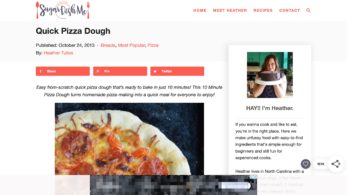**Descriptive Caption:**

This screenshot captures a webpage from the website "Sugar Dash Me," featuring a recipe titled "Quick Pizza Dough." The recipe, published in October (exact date unclear), is authored by Heather. The caption highlights the ease and speed of the recipe: "Easy, from-scratch quick pizza dough that's ready to bake in just 10-15 minutes. This 12-minute pizza dough turns homemade pizza making into a quick meal for everyone to enjoy." 

Heather's biography is prominently displayed on the right side of the page. It reads, "If you want to cook and like to eat, you're in the right place. Find easy-to-source ingredients and recipes simple enough for beginners while still fun for experienced cooks." She mentions living in North Carolina, though the bio cuts off there. Accompanying her biography is a picture of Heather proudly holding a chocolate cake.

Also displayed is an appetizing image of a freshly baked pizza, topped with pepperoni and cheese. The website includes options to contact Heather and explore additional recipes and features.